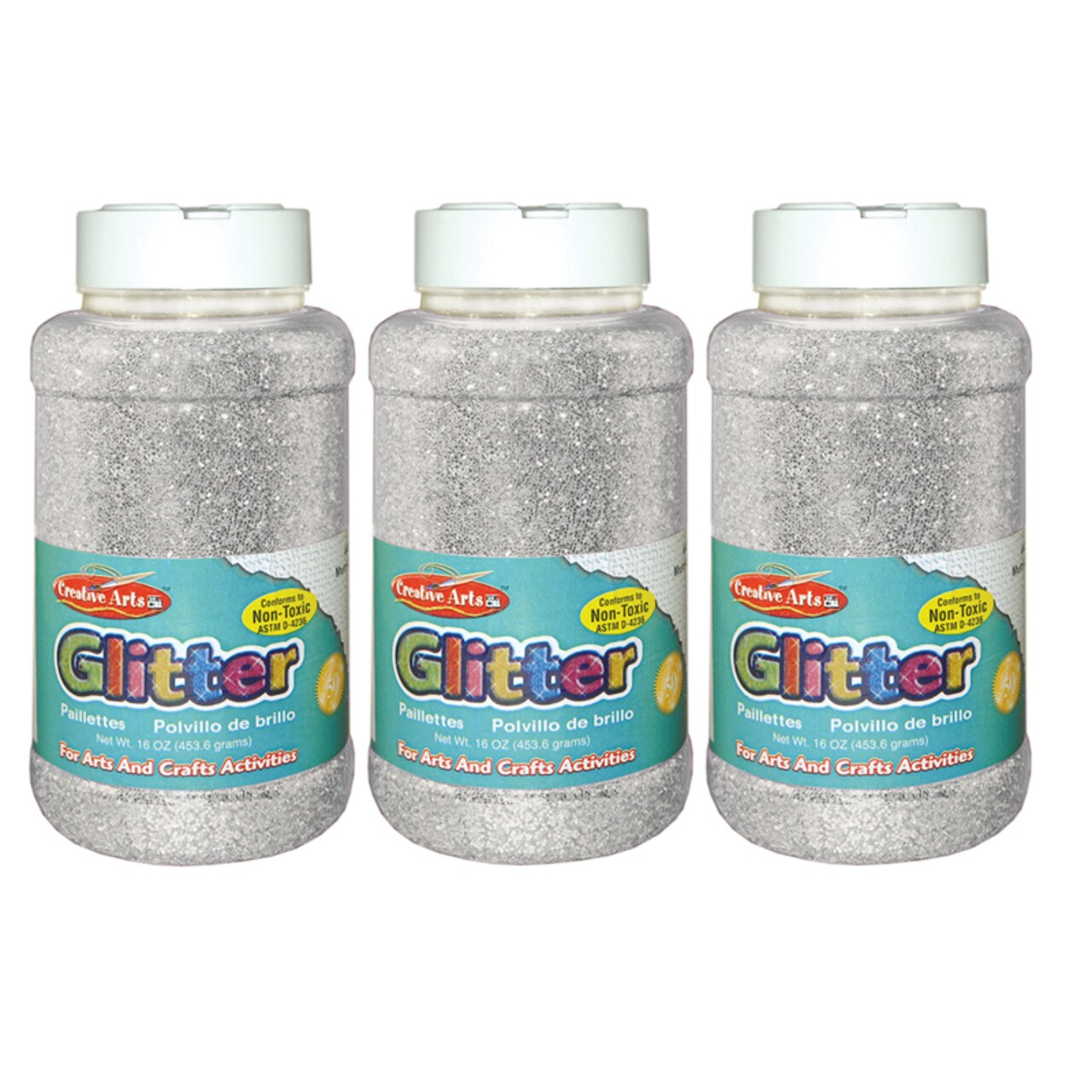The image shows three identical clear plastic bottles of Creative Arts non-toxic glitter, each containing 16 ounces of shimmering silver glitter. The bottles have clean, white caps and feature a detailed label with a teal-to-turquoise gradient background. At the top left corner of the label, there is a red oval with white text that reads "Creative Arts," with a paintbrush touching the 'i' in "Creative." In the top right corner, a yellow oval with black text states "non-toxic." The center of the label prominently displays the word "glitter" in large, multicolored letters, each letter filled with glitter of different shades—green, red, pink, yellow, blue, red again, and yellow again—outlined with blue and then white. At the bottom of the label, it specifies that the product is "for arts and crafts activities." The overall look is clean and vibrant, making these bottles visually appealing and suitable for artistic projects.